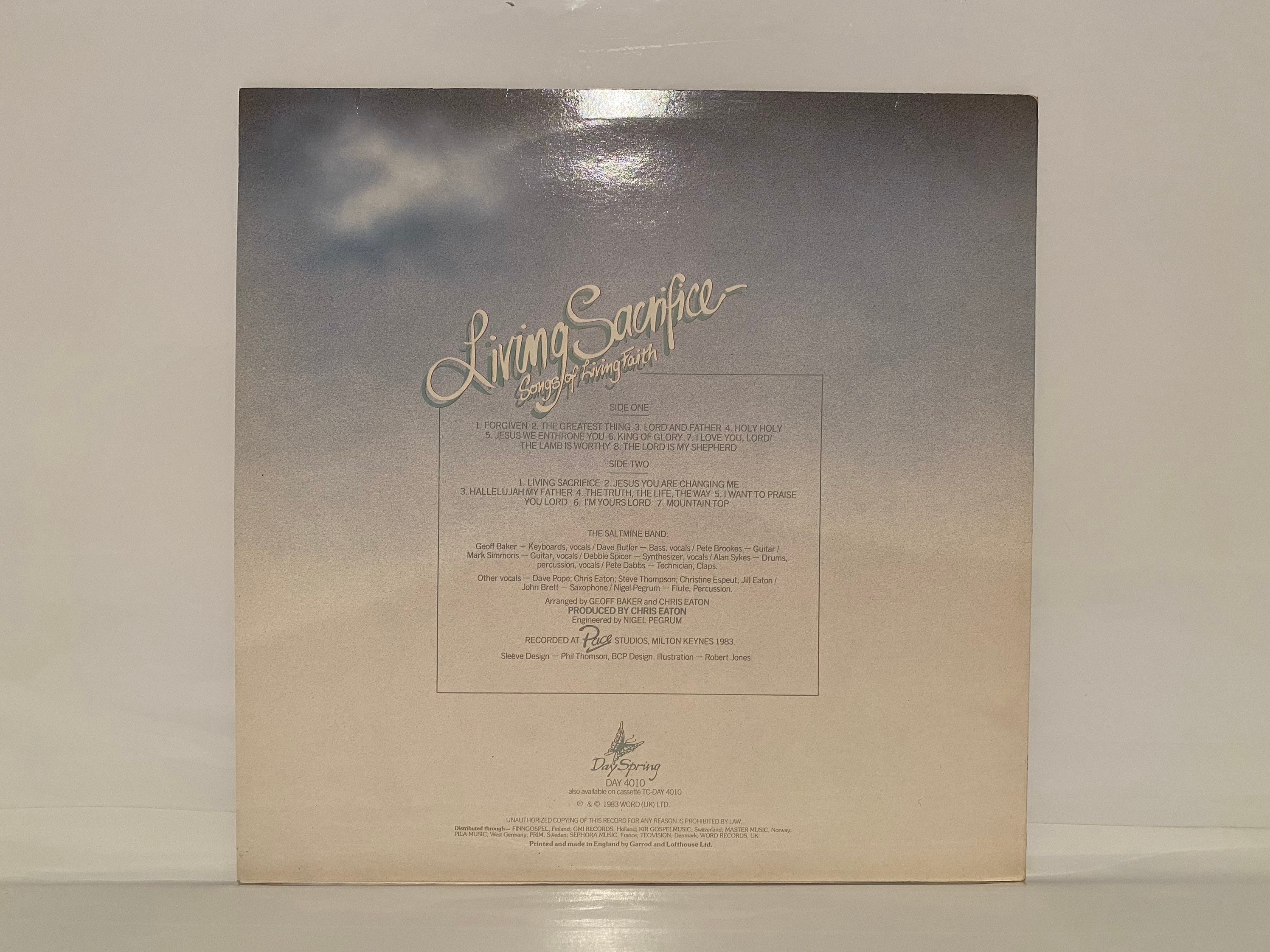The image depicts a photograph of a vintage music album leaning against a white wall and resting on a gray floor. The album cover features a blue-gray top half, resembling clouds, with a tan bottom half. A soft light reflection graces the top of the cover. In the middle, in a stylized cream-colored cursive font, the title reads "Living Sacrifice, Songs of Living Faith." A central black-outlined square lists the song titles for Side 1 and Side 2, with the names of the band members and recording information, including the venue, Pace Studio, and production by Dayspring in 1983. The arrangement credits go to Geoff Baker, and the production is by Chris Eaton. The overall aesthetic and text style hint that it is a religious worship or gospel album, possibly mistaken for a CD, but more likely the back cover of a record.